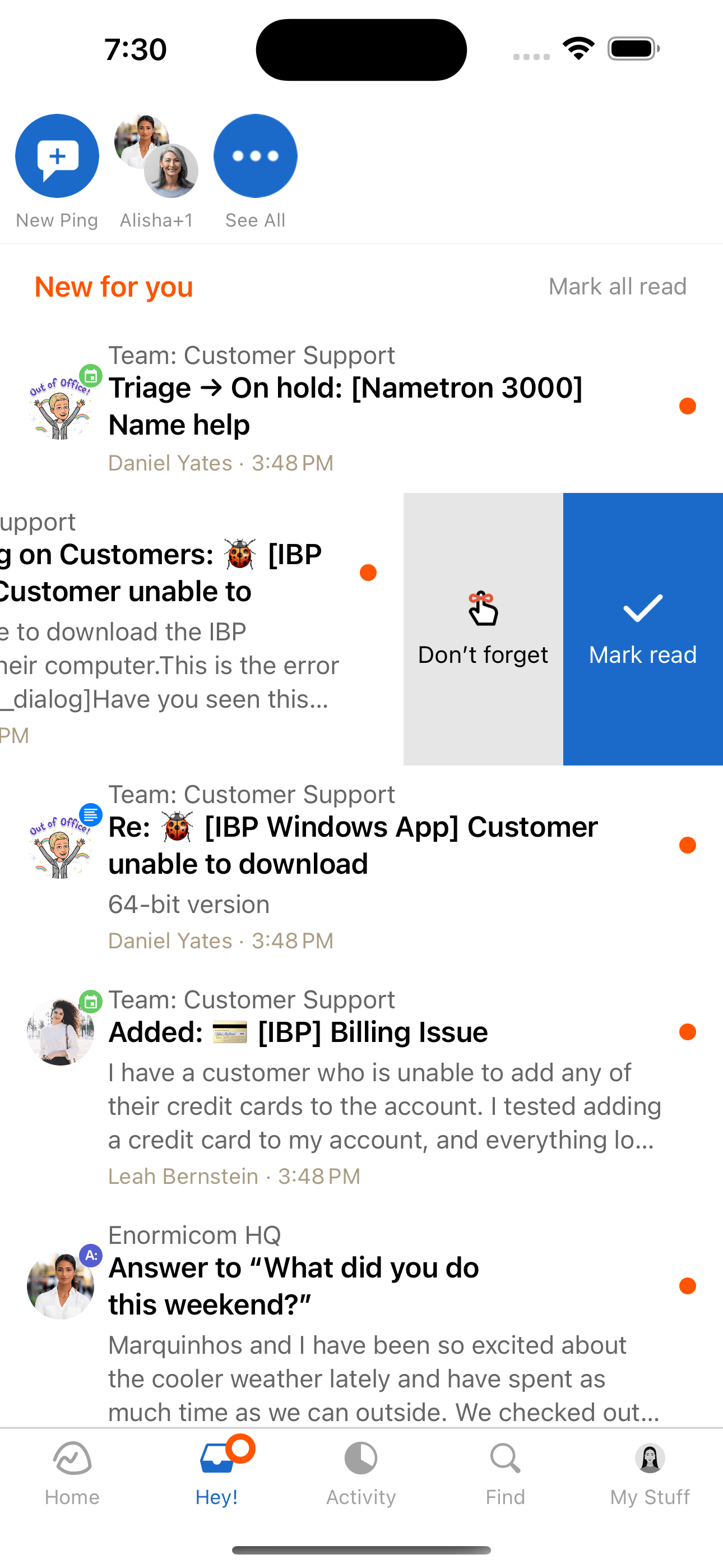**Detailed Caption:**

This screenshot captures a portion of a messaging interface. At the top center, there's a blue circle featuring a white speech bubble icon, labeled "New Ping." To the left of the "New Ping" label, two circular profile pictures of women are displayed with the text "Alicia plus 1" below them. To the right of the "New Ping" label, there is another blue circle containing three horizontal white dots. 

Directly below this section, the phrase "New for You" appears in orange text, with the option "Mark All Read" positioned to the right. 

Further down, there are various messages organized under different categories. The category labeled "Team" includes "Customer Support" and "Triage on Hold," with a bracketed description "name Tron 3000" and "name help."

In the lower section of the screenshot, another message displays two text areas on the right: a grey "Don't forget" section and a blue "Mark as Read" section placed directly beside it.